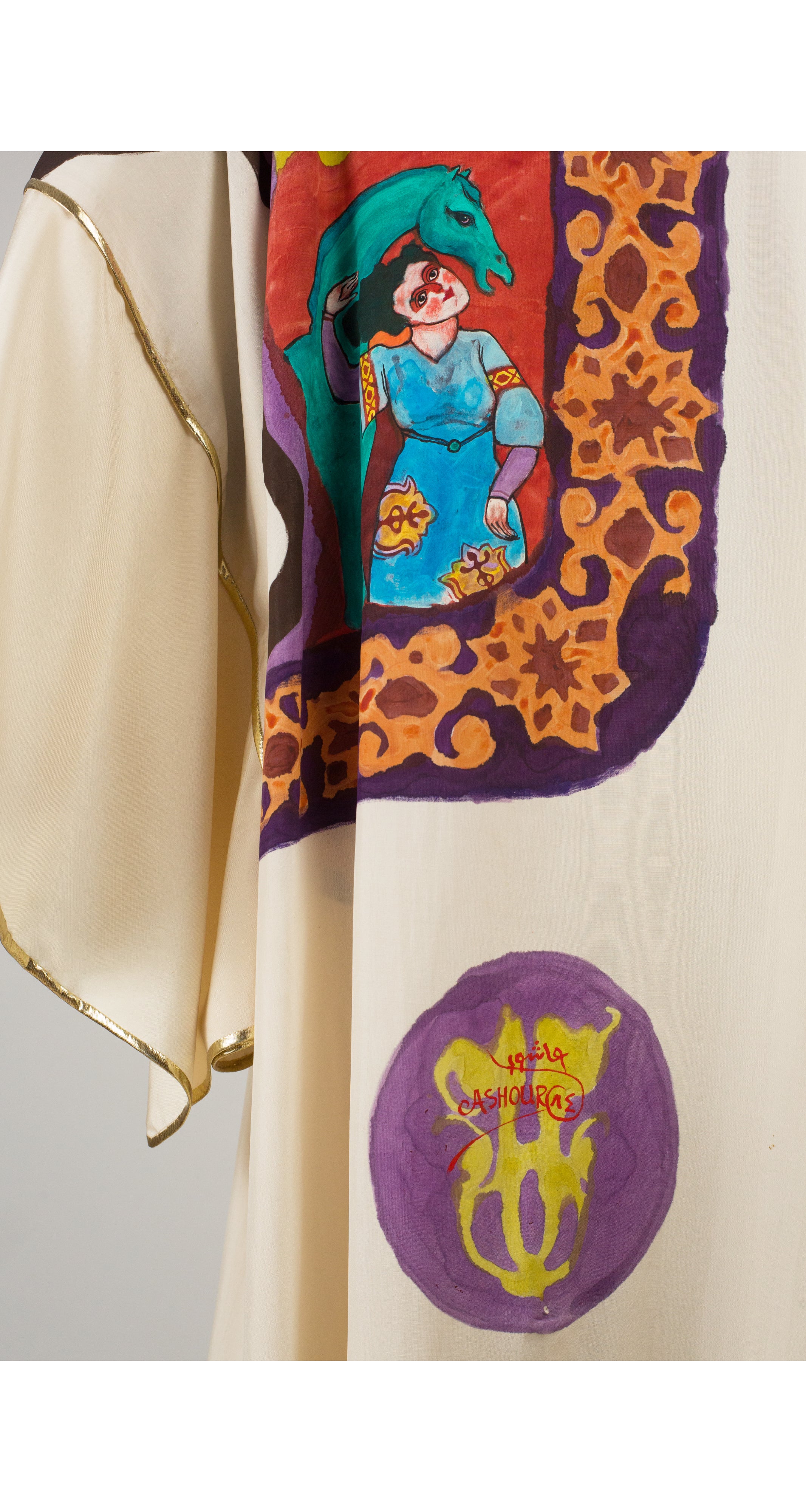This close-up photograph, taken in portrait layout, showcases a sumptuous white or cream-colored silk garment, possibly a robe or a costume, adorned with intricate details. The visible portion includes one sleeve and part of the torso, with thin gold fringes and seams outlining its edges, giving a luxurious touch. Prominently featured on the fabric is an ornate illustration depicting a dark-haired Caucasian woman with striking red eyes, donned in a blue dress embellished with gold and red accents. Beside her is a turquoise horse, set against a vivid red background. This scene is bordered by a rich purple band adorned with elaborate gold and brown designs. Beneath the illustration, the garment features a purple circle emblazoned with a golden crest or design, and adorned with unreadable red text, possibly in a foreign script. The overall depiction is rich in color, incorporating teal, blue, purple, orange, and violet hues, contributing to the garment's vibrant and opulent appearance.